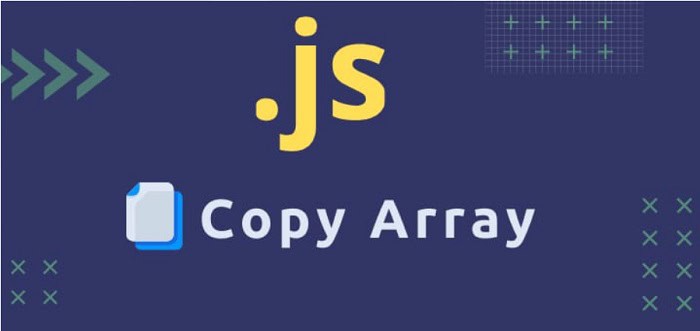A rectangular image features a purplish-blue background. On the left side, a series of green arrows point towards the right. Near the center, a prominent yellow circle is displayed with "JS" written in lowercase letters inside it. The background includes a grid formed by small white dots, interspersed with blue plus signs. Towards the bottom center, two overlapping pieces of paper are depicted: a white sheet with a dog-eared corner revealing blue underneath, and the text "Copy Array" written below. Four green X's create a square shape adjacent to the papers. On the right side, a column of four similar green X's runs vertically from top to bottom. The grid's dots and plus signs transition from whitish at the top to greenish in the middle and bottom areas.